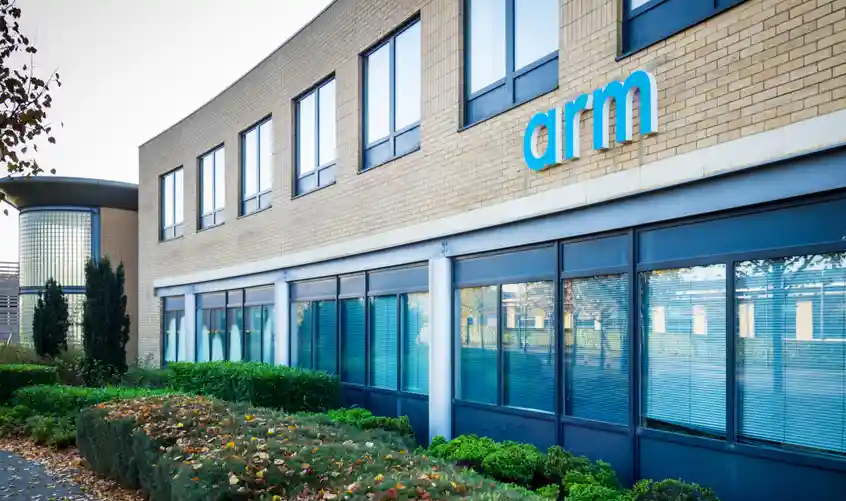This photograph captures a two-story office building featuring a beige brick facade above a series of black windows with white and silver borders on the bottom. The building is angled into the distance towards the left-hand side of the image, providing a full view of its front wall. Prominently displayed in blue letters on the side of the building is the word "ARM." The windows have tinted blue trims with drawn white blinds, reinforcing the office-like atmosphere. The lower part of the building is characterized by equidistantly placed concrete posts and numerous windows. In front of the building, there are green shrubs and low hedges adorned with fallen autumn leaves, adding a touch of seasonal change. To the far left, a cylindrical structure with a glass-tiled exterior and resembling a decorative entrance adds architectural interest. In the distance, some trees are visible, further contributing to the scene's depth. The overall ambiance is professional and quiet, with no people in sight.